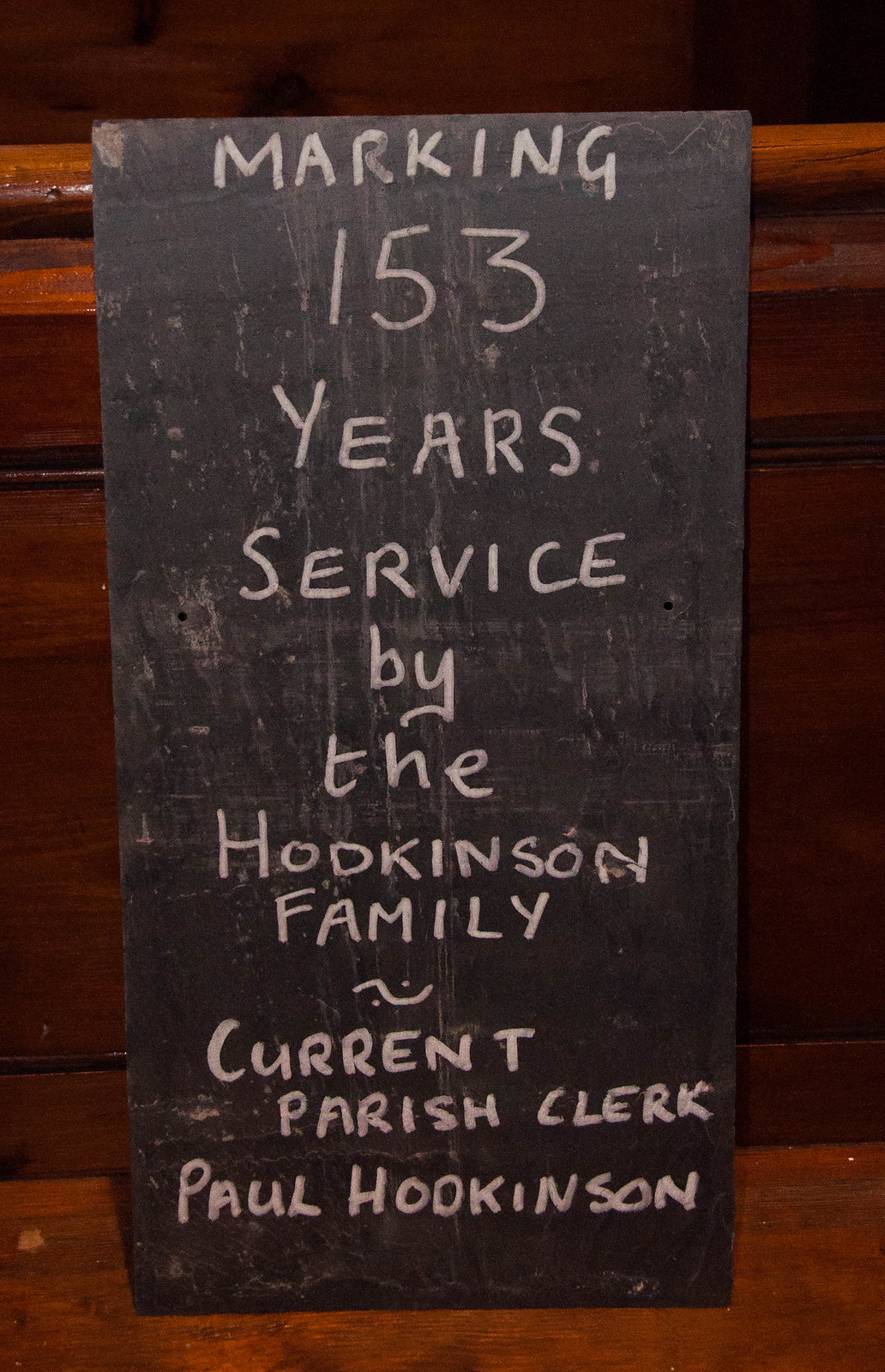The image depicts a rectangular, well-worn slate chalkboard standing vertically and centrally against a distinct wooden background that resembles a bench or banister, rich in brown and orange hues with visible wood grains and molded edges. The chalkboard, appearing damaged with smears, drip marks, and a chip on the upper left corner, bears a handwritten message in white chalk. The message, written in capital letters, commemorates "Marking 153 years service by the Hodkinson Family," with a squiggly line followed by "Current Parish Clerk, Paul Hodkinson." The scene is likely set indoors, perhaps in a restaurant or similar establishment.